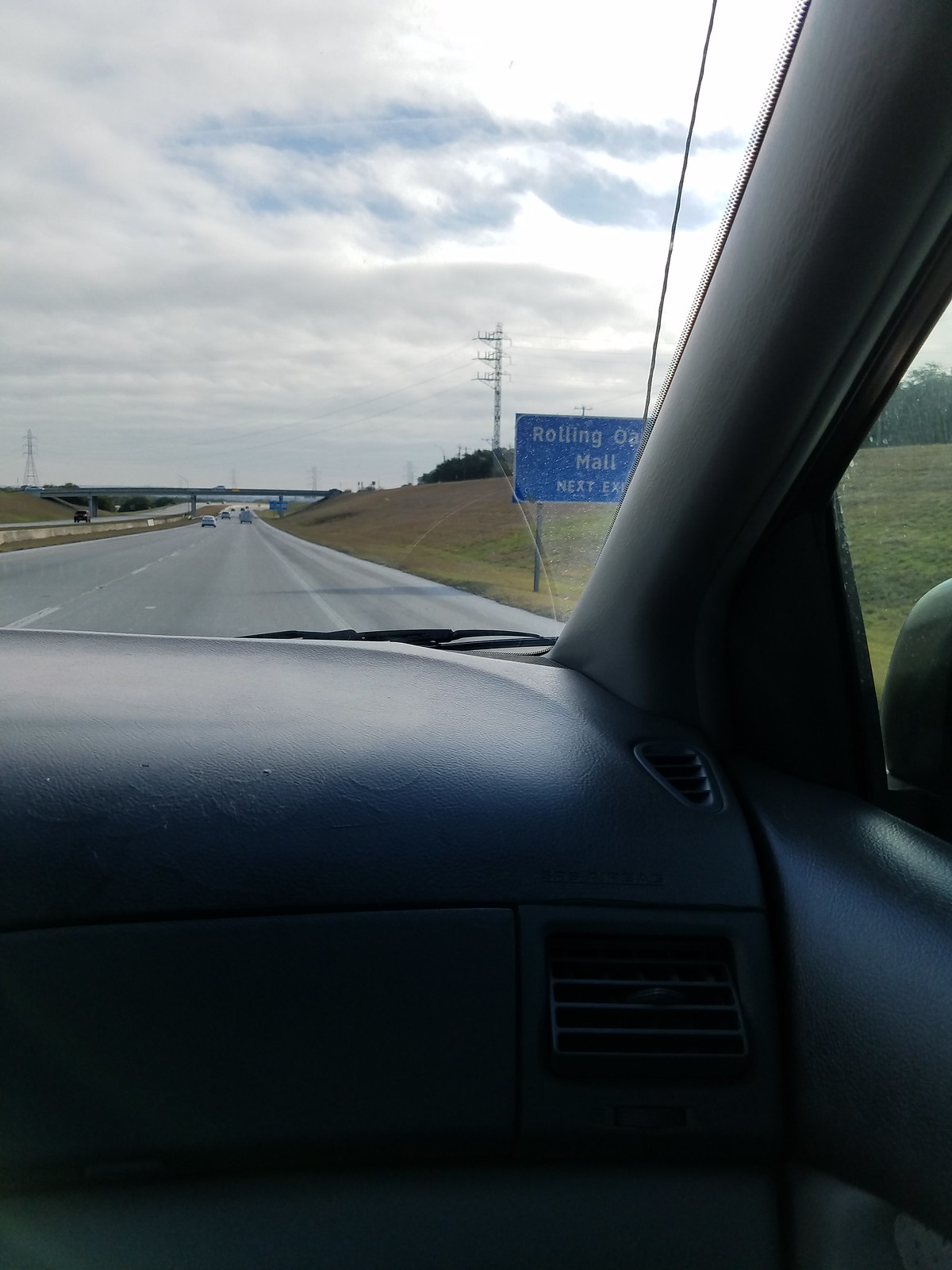A detailed car interior and highway landscape: The photograph captures the interior of a car from the perspective of the passenger seat, showing the right side of the cabin including part of the dashboard and the passenger-side mirror. Beyond the car's window, a four-lane highway stretches ahead, separated by a grassy median. An overpass is visible in the distance, beneath a sky filled with fluffy white clouds, indicating daytime. To the right of the highway, there's a shoulder, which leads to a dry, grassy, hilly area. A blue street sign reads "Rolling Something Mall Next Exit" in white text. In the background, an electricity pole stands, hinting at the infrastructure that supports the area.